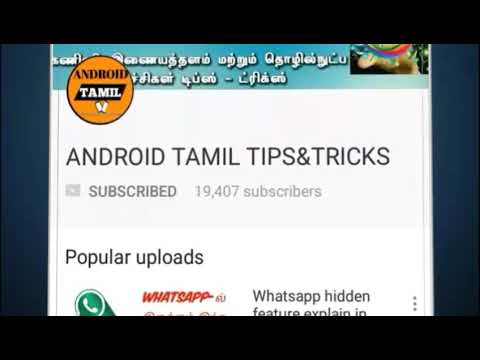This image appears to be a screenshot from a webpage or social media page that offers videos, specifically focusing on tips and tricks for Android in Tamil. The image is bordered at the top and bottom with black strips, which have a blueish tint towards the edges. In the upper left corner, there is an orange circle containing the text "Android" in black and "Tamil" in white with a black background. Adjacent to this, a blue rectangular banner features foreign text in white. Below the banner, the main title "Android Tamil Tips and Tricks" is prominently displayed in black font. The text "Subscribed" appears in dark gray, with "19,407 subscribers" written in lighter gray to the right of it. The section titled "Popular Uploads" is followed by an entry labeled "WhatsApp," which is bolded and italicized in red font. Below this, the phrase "WhatsApp hidden features explained in" is written in black font. A green circle with a white telephone symbol and a surrounding white ring also appears below this text. In the upper right corner, there's an unclear image resembling a red dog collar or possibly a turtle, with something brown and possibly leafy beneath it.